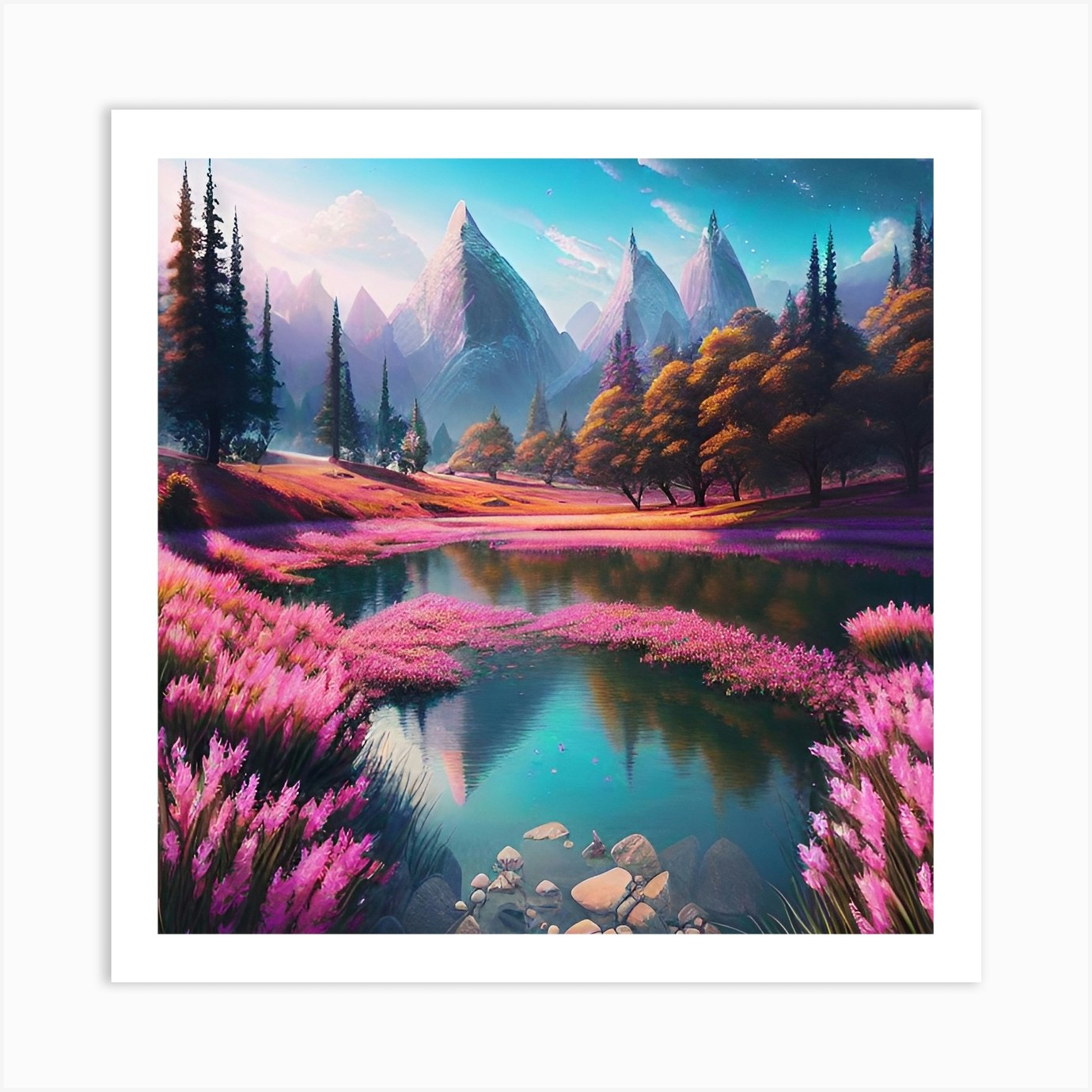This vibrant digital artwork, displayed in a thick white frame, presents a picturesque mountainous landscape characterized by vivid colors and intricate details. Dominating the background are towering, jagged mountains, their peaks dusted with snow and shaded in hues of pinks and purples. Above, a clear blue sky dotted with cloudy formations casts a serene ambiance over the scene. Descending from the mountains, the terrain transitions into rolling hills adorned with a variety of trees: tall pine trees, fluffy-leafed trees, and brown and golden amber foliage.

In the foreground, a tranquil blue lake with reflections of the bright sky and mountainous peaks stretches across the scene. Around this lake, an abundance of pink flowers in various shades — light pinks, dark pinks, and mauves — create a vibrant border, some even floating delicately on the water's surface. Strategically placed rocks punctuate the lake's expanse, adding depth and texture to the peaceful waterscape. The composition's rich palette of pinks, blues, greens, and earth tones collectively evokes a sense of serenity and natural beauty.